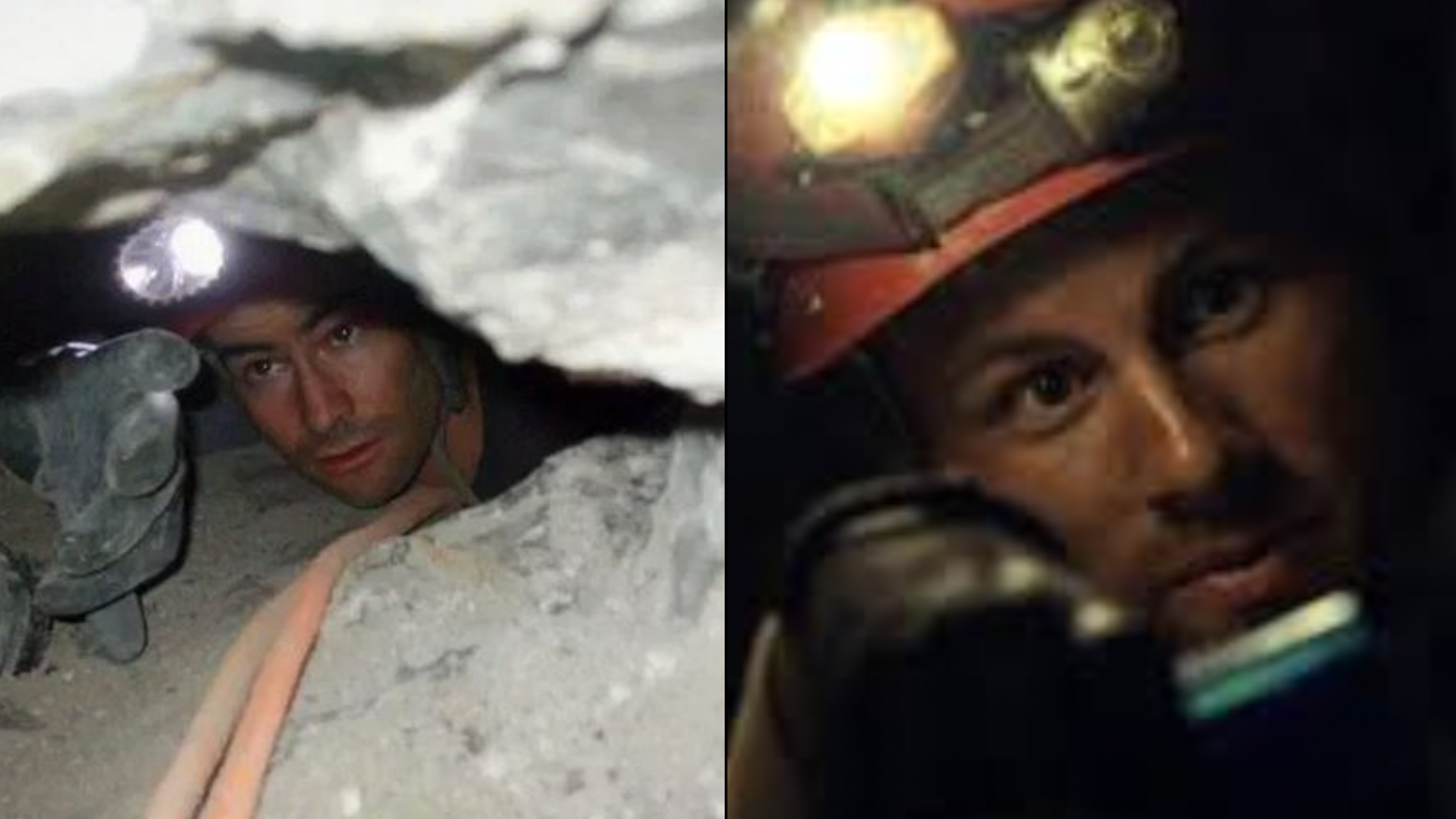The split-screen image captures two side-by-side photographs of what appears to be a cave explorer or scientist. On the left side, a man with a five o'clock shadow, wearing a helmet equipped with a headlamp, peers through a narrow crevasse. The dimly lit cave around him reveals gray and white rock formations, and ropes are visible, possibly tied to him for safety. On the right side, an up-close view of the same man shows him looking directly into the camera with his headlamp turned on. The dark background envelops him, making the illuminated parts of his gear and face stand out starkly. Under his lips, there is a blue and white object, which might be the handle of two toothbrushes, though it's not clearly identifiable. The overall image depicts the intensity and solitary nature of cave exploration, enhanced by the surrounding darkness.